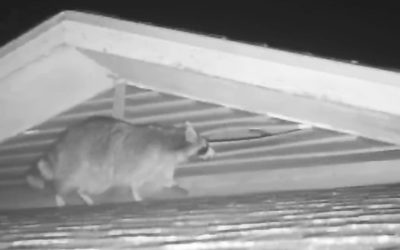This black-and-white night vision image appears to have been captured by a security camera. It shows a raccoon in a close-up, angled frame as it walks across the shingles of a rooftop. The raccoon is depicted in profile, moving towards the right side of the image. Its distinctive striped tail and the mask-like markings on the right side of its face are clearly visible. The background is dark, indicating it is nighttime. In the foreground, the angled portion of the roof is visible, featuring shingles and a white overhang with wooden slats that slope downward. The raccoon is positioned slightly toward the left side of the image, enhancing the sense of movement. Its eye appears white, likely reflecting the camera's infrared light or laser. This scene suggests the use of a motion sensor to trigger the camera.